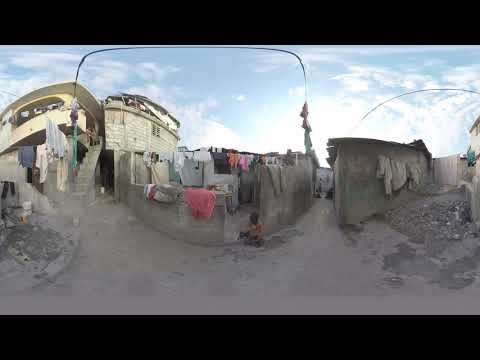The image presents a heavily distorted, 360-degree view of a small, impoverished village, imparting a disorienting fisheye effect. At the center, there is a dusty, narrow alleyway bordered by concrete and stone walls, some appearing ancient and in disrepair. The area looks rundown, with several small, dilapidated buildings—some resembling mere shacks—scattered throughout. The ground is a brownish-gray dirt, adding to the overall bleak atmosphere. 

A cream-colored wooden building with a stone staircase leading up to it stands prominently on the left. Laundry—scrappy and varied in colors such as pink, white, gray, yellow, and green—drapes over walls and hangs from lines strung between the buildings, reflecting the residents' modest means. 

In the doorway of one concrete structure, a little black boy in an orange top is playing, though the image's out-of-focus quality makes his features indistinguishable. Behind him, a taller stone structure looms, contributing to the cluttered skyline, and beyond it, the sky is a bright blue with scattered white clouds, with the sun's bright white light casting an intense glare from the right side of the photograph.

Amidst the dusty streets and worn-out infrastructure, the village's state of poverty is starkly evident, capturing a poignant snapshot of its harsh living conditions.